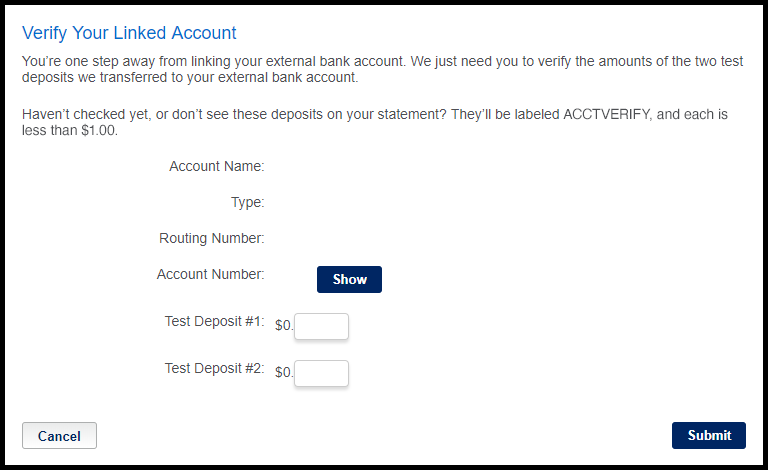The image is a screenshot of a verification screen for a website. At the top left, the header displays in blue text: "Verify Your Linked Account." Beneath the header, it states, "You're one step away from linking your external bank account. We just need you to verify the amounts of the two test deposits we transferred to your external bank account." Following this, there is an advisory message explaining, "Haven't checked yet or don’t see these deposits in your statement? They’re labeled ACCTVERIFY (in all caps), and each is less than $1."

Further down, the form requires specific details with labeled fields for "Account name," "Type," "Routing number," and "Account number." Next to the "Account number" field is a dark blue button labeled "Show" in white text, which presumably reveals the account number when clicked.

Below these fields, the form requests the user to input the exact amounts of the test deposits. The first entry field is labeled "Test Deposit Number One," followed by a field marked "0.XX," indicating space for the user to enter the first deposit amount. Similarly, "Test Deposit Number Two" follows, with another entry field labeled "0.XX" for the second amount.

This verification process ensures the user's bank account is securely linked to the platform by having them confirm the small deposit amounts transferred to their bank account. Once the user verifies these amounts, the account linkage is confirmed, allowing secure transactions to proceed seamlessly.